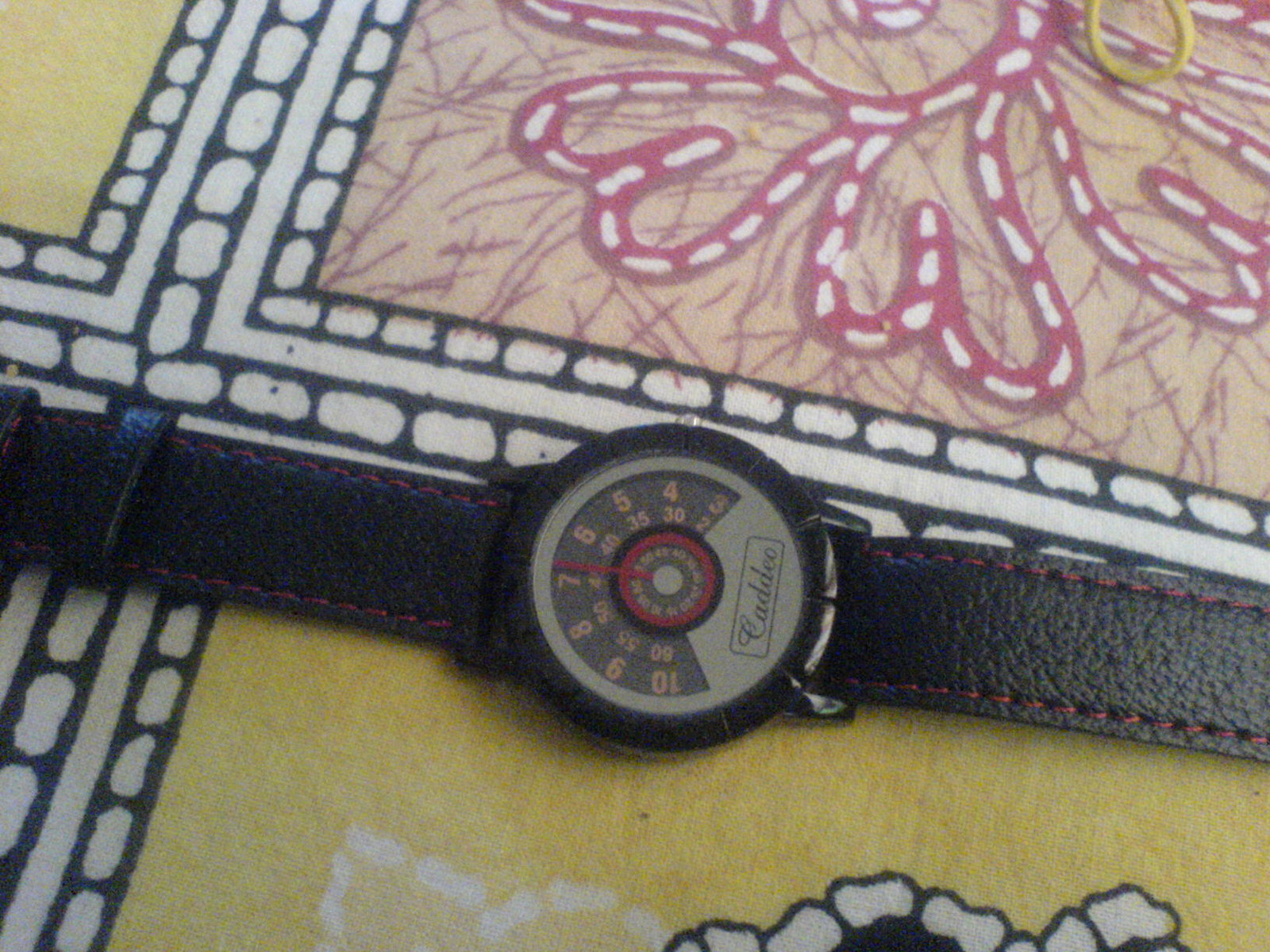This detailed photograph captures a stylish watch positioned on a vibrant, multicolored surface comprising a grid-like pattern of squares. Each square is delineated by black borders, with solid and dashed white lines adding to the intricate design. The pattern includes a mix of colors, where one square features light brown, red, and white hues, while another displays a combination of yellow, black, and white.

The centerpiece of the image is the watch, which boasts a black band adorned with striking red stitching. The watch’s bezel is also black, creating a bold contrast against its light gray face. The brand name "Catio" is elegantly written in cursive at the bottom of the watch face. The design includes a half-circle arrangement of numerical markers to indicate the hours, a prominent display of the current time, and a smaller sub-dial dedicated to tracking seconds with a single hand. This composition highlights the watch's sophisticated design against an eye-catching backdrop, offering a blend of modern aesthetic and functional elegance.